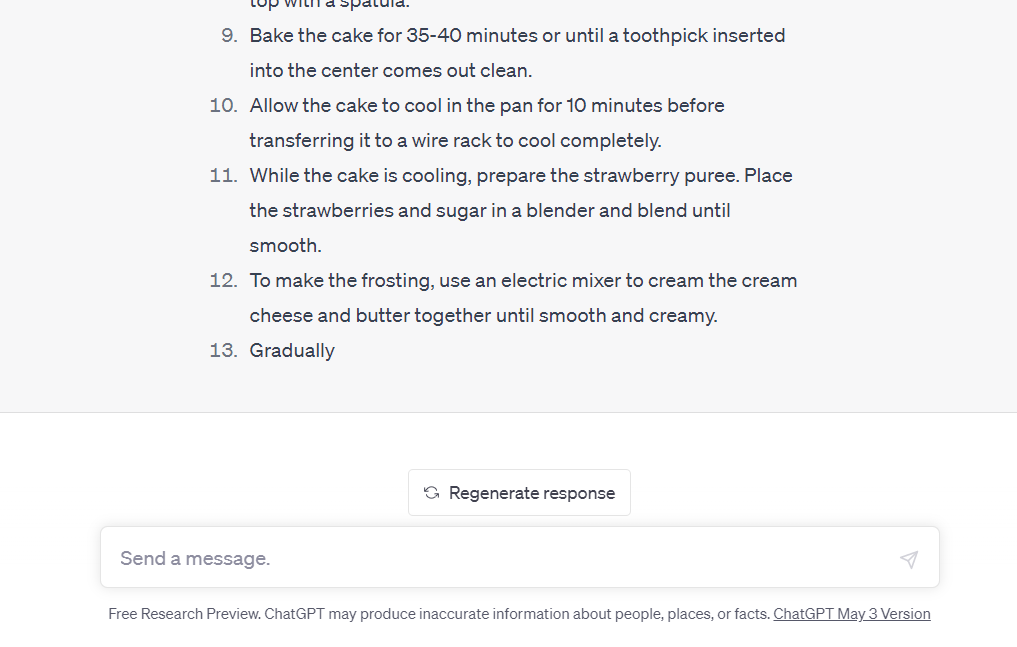After baking the cake for 35-40 minutes, or until a toothpick inserted into the center comes out clean, let it cool in the pan for 10 minutes. Then transfer the cake to a wire rack to cool completely. Meanwhile, prepare the strawberry puree by blending strawberries and sugar until smooth. For the frosting, use an electric mixer to cream together cream cheese and butter until smooth and creamy.

---

In the kitchen, a deliciously moist cake, freshly baked to perfection, is cooling on a wire rack. After 35-40 minutes in the oven, and a successful toothpick test, this cake now awaits its sweet, tangy strawberry puree and a rich, creamy frosting. The luscious puree is crafted by blending ripe strawberries with sugar until silky smooth. Nearby, an electric mixer is effortlessly blending cream cheese and butter into a velvety frosting, ready to generously coat the cake once it’s fully cooled. The detailed preparation showcases the dedication and love put into creating this delightful dessert.